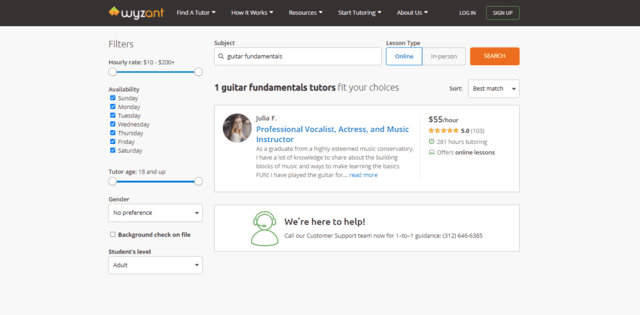This is a detailed caption for an image featuring a website screenshot:

The website screenshot displays Wyzant's homepage. The top banner features a black background with a chevron-style logo in the upper left corner – green at the top and orange at the bottom – accompanied by the brand name 'Wyzant' (W-Y-Z in white and A-N-T in orange). The navigation bar includes clickable options: 'Find a Tutor,' 'How It Works,' 'Resources,' 'Start Tutoring,' and 'About Us.' To the right, there are two buttons: a white 'Log In' button and a green-bordered 'Sign Up' button with white font.

To the left, on a white background, there's a sidebar featuring filter options. The filters include 'Hourly Rate' (ranging from $10 to $200+), 'Availability' with blue check marks for each day of the week, 'Tutor Age' (18 and up), 'Gender' (no preference), and an unchecked 'Background Check on File.' Further filtering options are 'Student Level' (adult), 'Subject' (Guitar Fundamentals), and 'Lesson Type' (online or in-person, with online highlighted). An orange 'Search' button is below these filters.

The main content area highlights a tutor matching the selected filters. It features an image of a young woman with blonde hair, identified as Julia F. She is described as a professional vocalist, actress, and music instructor who graduated from a highly esteemed music conservatory. Julia offers to share her knowledge on the building blocks of music and fun ways to learn the basics. Her profile includes a rate of $55 per hour, a perfect 5-star rating from 103 reviews, 281 hours of tutoring experience, and an option for online lessons.

A final note at the bottom offers customer support contact: "We're here to help. Call our customer support team for one-on-one guidance at 312-646-6365."